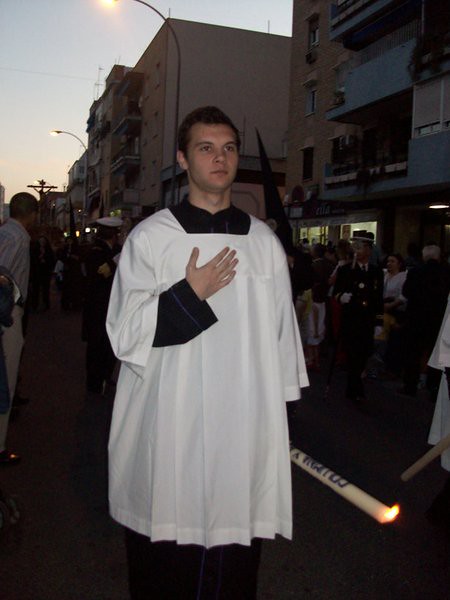In this image, a religious figure, possibly a Catholic priest or brother, is depicted walking through a crowded street during a religious parade or event. It is early evening, and the sky is transitioning from blue to dark, creating a dusk ambiance. The priest is distinguished by his white tunic with a black shirt underneath and has dark hair. He is holding a white, lit object—potentially a candle or a torch—with blue writing on it, which is difficult to discern. His left hand is placed over his heart, suggesting he might be praying. In the background, several four-story brick buildings line the street, which seems busy with many onlookers standing on either side. To the left, a raised crucifix is faintly visible against the darkening sky. Additionally, one person in the crowd to the right appears to be dressed in white gloves and attire resembling a military or police uniform. The overall scene reflects a solemn, community-focused event set against the backdrop of a bustling urban environment.